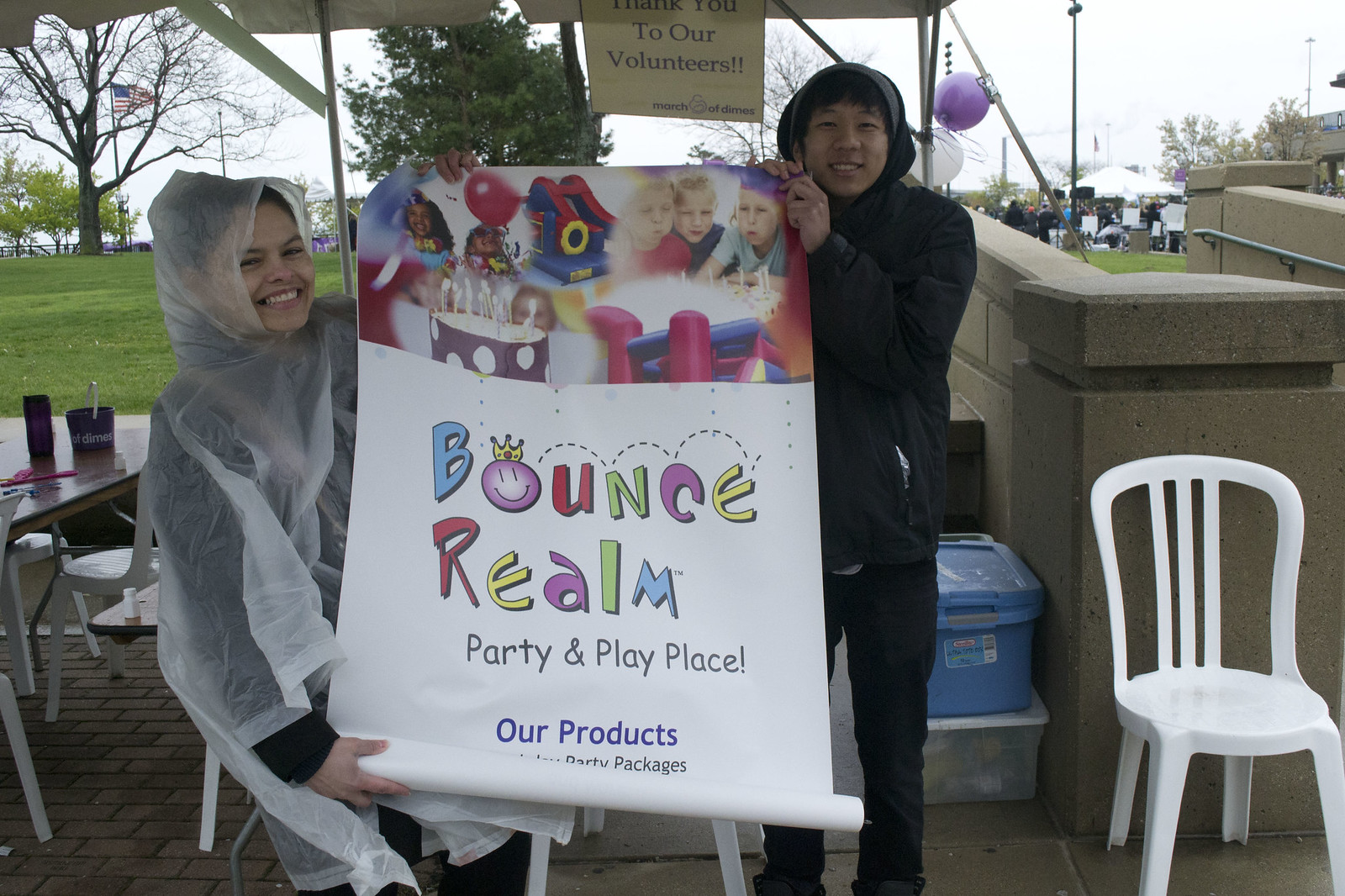In this outdoor, daytime photo, possibly taken in the rain, a woman and a man are prominently featured holding a colorful poster amid a setting that blends natural and urban elements. The woman, clad in a see-through rain poncho over her clothes, and the man, dressed in a black hoodie, both appear to be either Asian or of Hispanic descent. They stand on a mix of brick and tile flooring, with a green, grassy park extending into the background. Their poster, adorned with an image of children at a birthday party, reads "Bounce Realm, Party and Play Place, Our Products" in a vibrant, playful font.

A variety of details frame the scene: to the right of the man, a plastic chair sits nearby, and directly behind him is a blue storage container. Behind the woman, more chairs and a table with a cup are visible. A sign in the background expresses gratitude with the words "Thank You to our Volunteers." Additional elements include a park featuring lush greenery, trees, an American flag, traffic poles, and scattered groups of people in the distance. The overall scene is bustling yet intimate, capturing a small gathering under overcast, rainy skies.